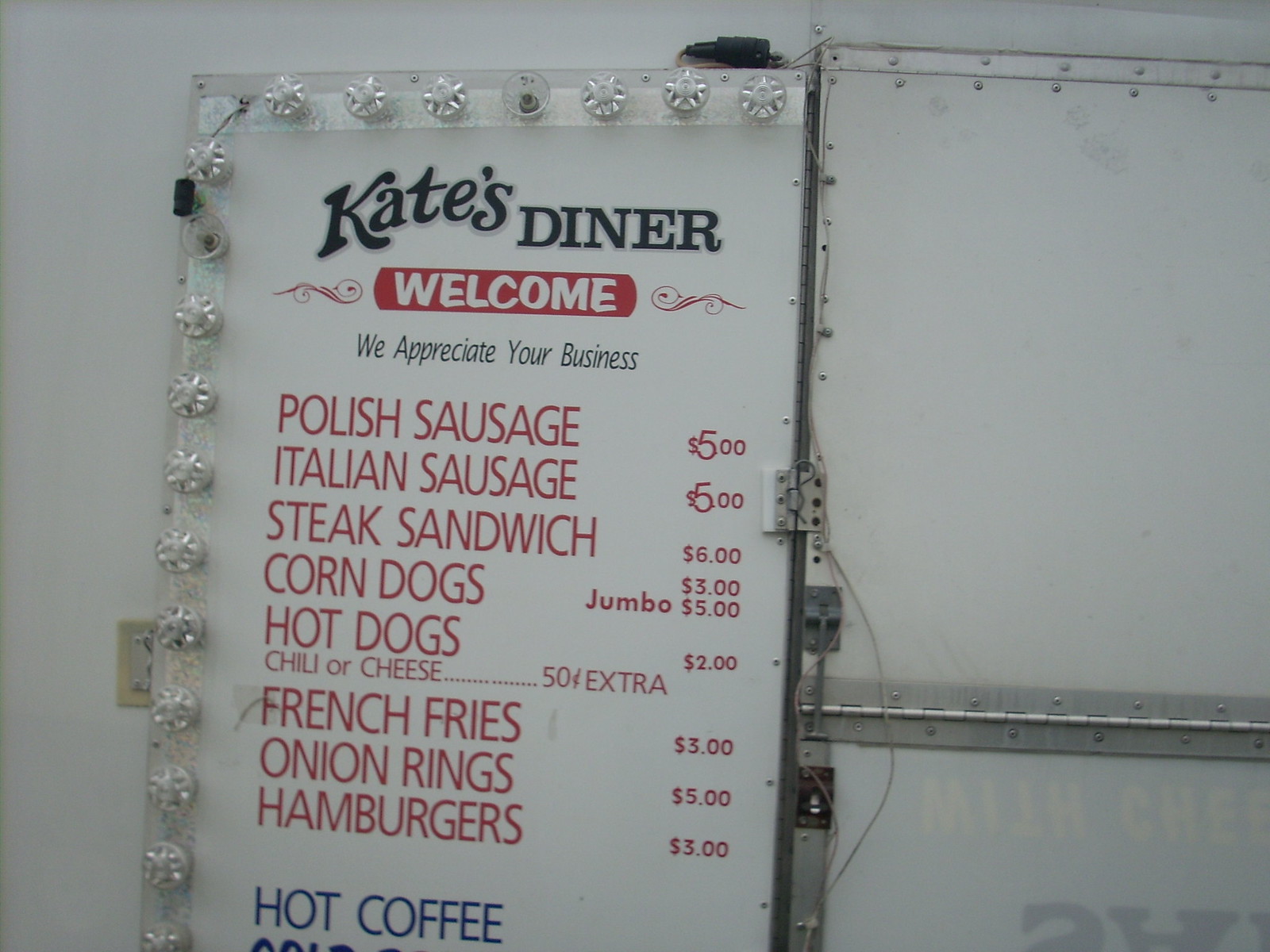The photograph, taken indoors, features a central white menu board titled "Kate's Diner: Welcome, We Appreciate Your Business." The board, adorned with decorative borders possibly illuminated by lights, lists menu items in red text, with the prices aligned to the right. The items include:
1. Polish sausage - $5.00
2. Italian sausage - $5.00
3. Steak sandwich - $6.00
4. Corn dogs (jumbo) - $5.00
5. Hot dogs - $2.00 (with chili or cheese for an extra $0.50)
6. French fries - $3.00
7. Onion rings - $5.00
8. Hamburgers - $3.00

Beneath these, in blue text, "Hot coffee" is listed. The menu is set against a white wall, with visible wires, nuts, and bolts on the sides.